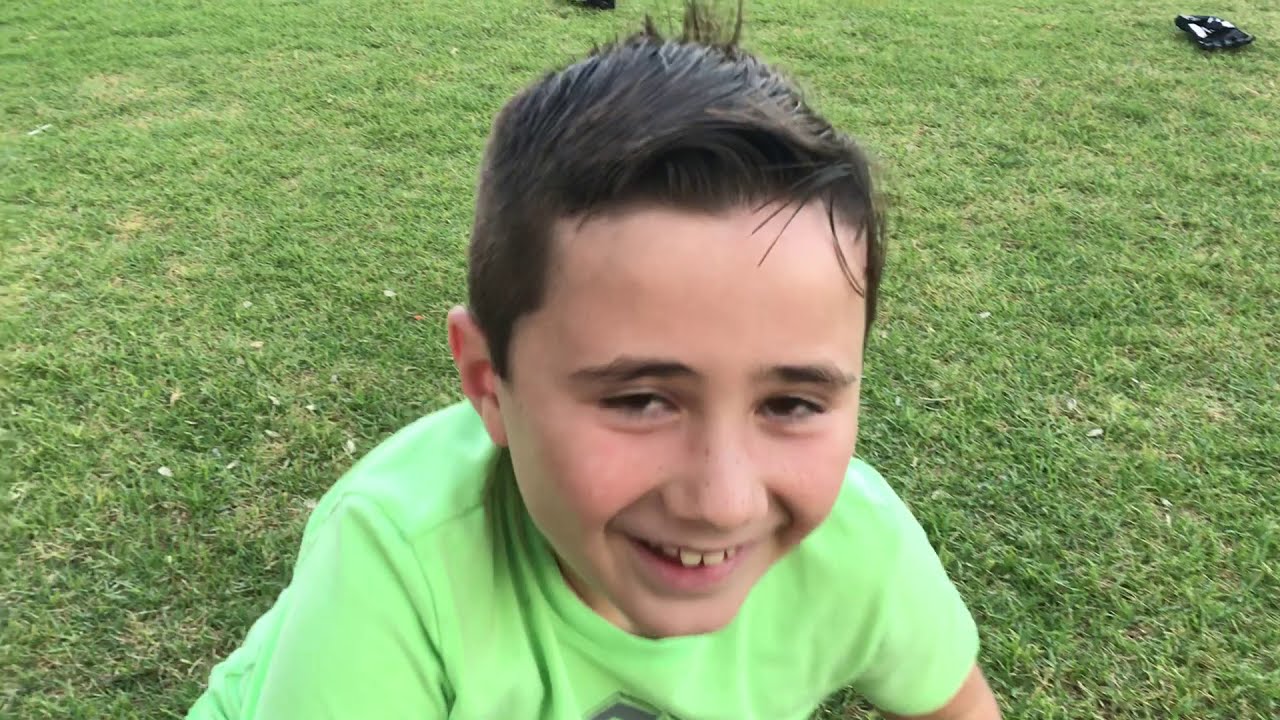The image is a close-up shot of a young boy with light skin and dark brown hair. His hair is slightly messy, with some gelled spikes at the back. He wears a light green T-shirt and smiles brightly at the camera, showing his teeth. His eyes are partially open, gazing slightly to the left. The background features a lush, green grass field reminiscent of a pristine golf course, indicating a well-maintained outdoor setting. Though the focus is on his face and the top of his shoulders, a baseball glove is visible on the far right edge, suggesting he might be enjoying a game of catch on a sunny summer day. The vivid green grass around him enhances the lively and playful atmosphere of the photo.